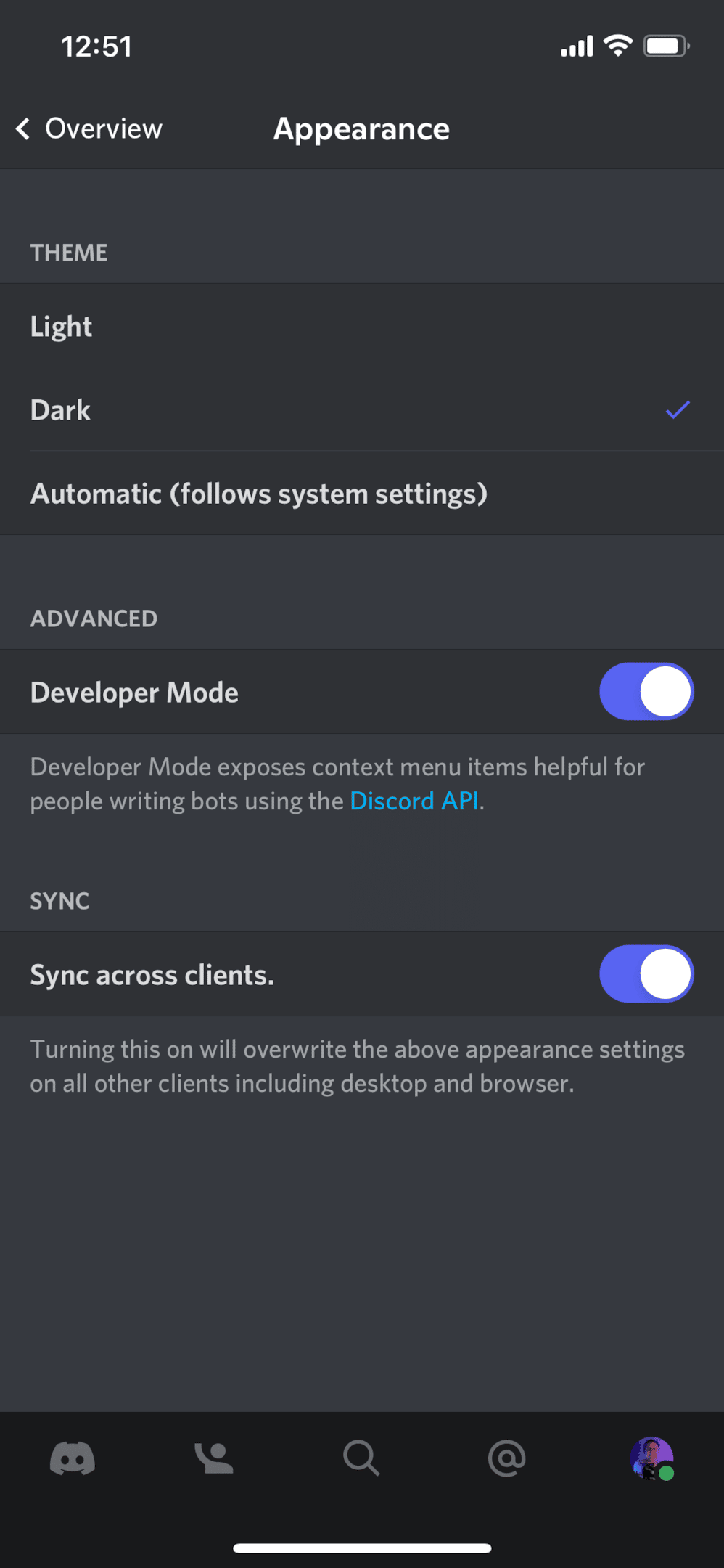Screenshot of Discord App on iPhone Showing Appearance Settings

This screenshot, captured at 12:51 PM, showcases the Appearance Settings page within the Discord app on an iPhone. The standard iPhone status icons – signal strength, Wi-Fi, and battery life – are visible at the top right corner. To the left, an arrow allows navigation back to the Overview page.

In the center, the title "Appearance" is prominently displayed above a dark gray background containing various options listed in rows with light gray text. These options include:

- **Light**, **Dark**, and **Automatic** (follows system settings).

Further down, an **Advanced** category is present, featuring:

- **Developer Mode** which is toggled on. This mode enhances context menus and menu items, particularly useful for those writing bots using the Discord API.
- **Sync Across All Clients**, also toggled on. Turning this on will synchronize appearance settings across all devices, including desktop and browser clients.

At the bottom, typical navigation icons are displayed alongside the user's avatar, although details of the avatar are not distinguishable. The icons include:
- The Discord logo for the home page
- A person raising their hand for mentions
- A magnifying glass for search
- An at symbol for mentions and replies

This detailed screenshot provides a comprehensive view of the customizable Appearance Settings available on the Discord mobile app.